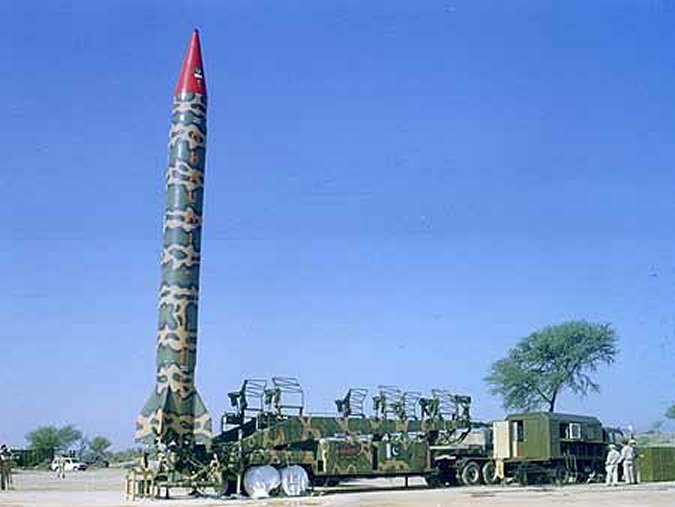The photograph presents a detailed scene of a section of an army base featuring a prominently displayed mobile rocket. The missile, positioned on the left side of the landscape-oriented image, stands upright on its base with a slender, cylindrical body painted in camo green and a pointed red nose cone. Intricate designs are visible along its body, and there appears to be an image resembling Daffy Duck on the nose.

Beneath the missile, which has flared fenders extending from its base, is a camo-patterned tractor trailer used for transport. This vehicle's dark green cab is situated at the bottom right of the image. Adjacent to the rocket setup is a small, compact mobile home or office space, contributing to the operational feel of the setting.

The scene captures the presence of several individuals dressed in white uniforms, scattered around the periphery, suggesting activity and readiness. A couple of additional vehicles are parked nearby. The setup with seats around the trailer, although seemingly risky due to the rocket's proximity, hints at possible observational purposes. The overall image, rich in representational realism, is detailed and vibrant, emphasizing the functional and military character of the environment.